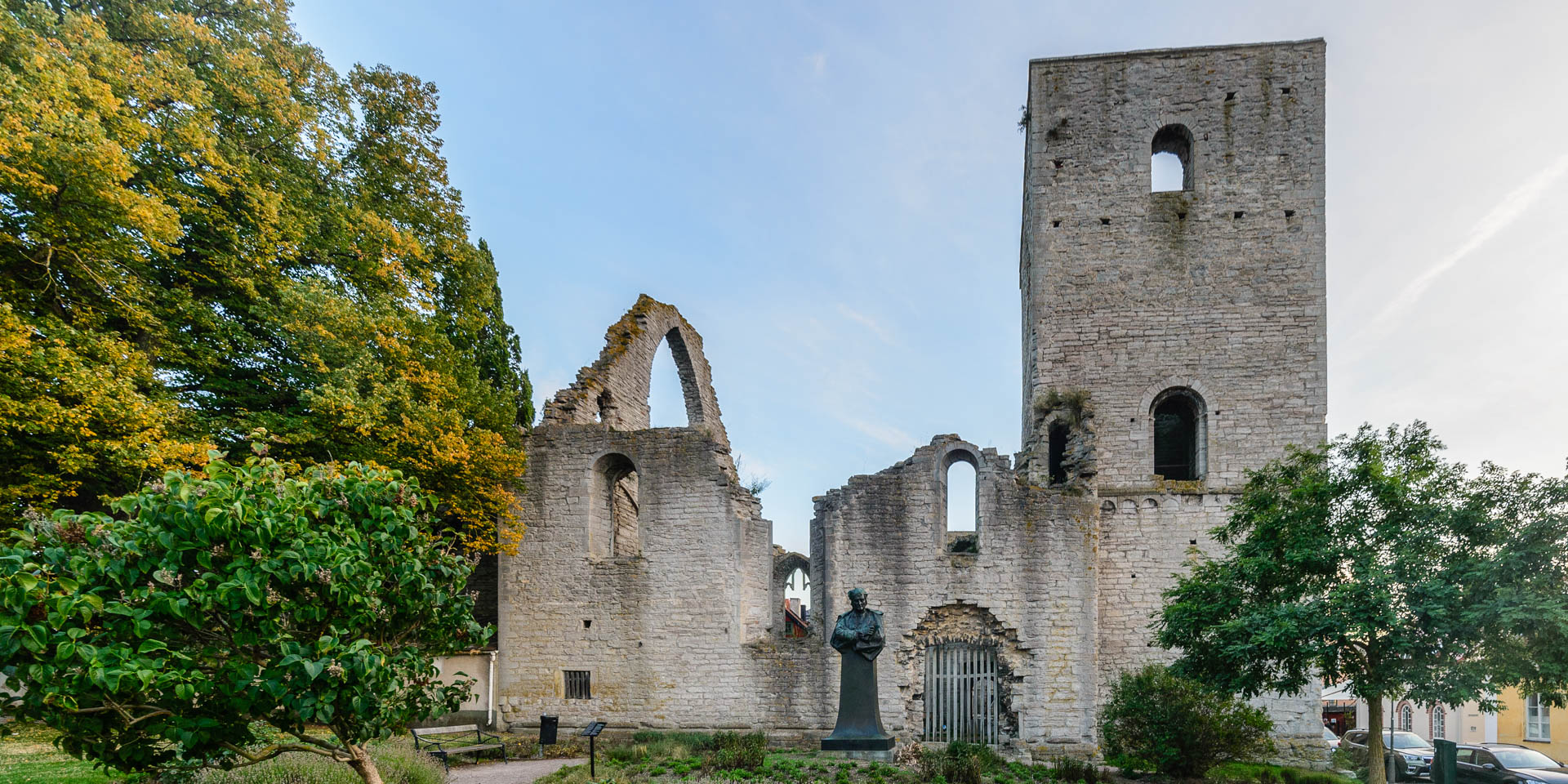The image depicts a historical gray brick building reminiscent of an old-world castle or possibly an ancient church or monastery. The structure appears partially gutted, lacking a roof, and its windows are hollowed out, suggesting past fire damage or long-term neglect. Dominating the front entrance is a striking black statue of a man in a robe, standing beside a noticeable gate that resembles something you'd find on a prison cell. 

In the foreground, the scene features a modest bench and a podium, possibly providing information about the building. A large green tree juxtaposes the entrance to the right, under which a few cars are parked, indicating the photo was taken in the present day. On the left side, dense greenery with tall trees, some sporting yellow leaves, adds a natural frame to the setting. The sun brightly illuminates the scene, revealing a clear sky and casting vibrant daylight across the deteriorating yet authentically historical structure.